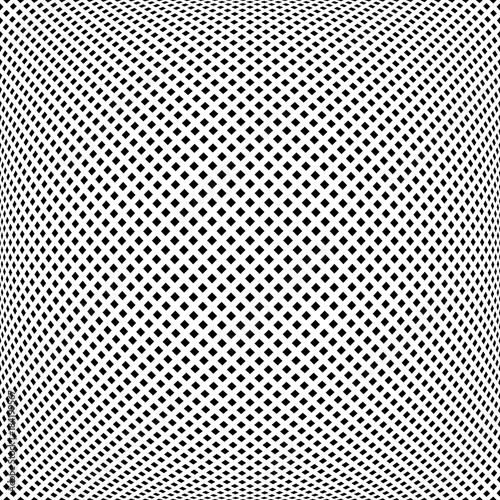This intricate optical illusion image features a white background with black squares that appear to transform into diamonds due to their diagonal alignment. The squares are larger at the center and gradually decrease in size towards the edges, creating a pattern that draws the viewer's eye to the middle, giving an illusion of depth and a 3D effect as if the center is popping out. The image is further complicated by blurred lines at the corners, enhancing its trippy, curving appearance. Bordering the black squares, the white spaces add contrast, intensifying the illusion. In the lower left corner, faint red text, possibly reading "Adobe Stock," is partially obscured by the overlaying squares, along with some unreadable numbers, suggesting an artist's signature or watermark. This detailed and dynamic composition makes the image captivating and visually engaging.